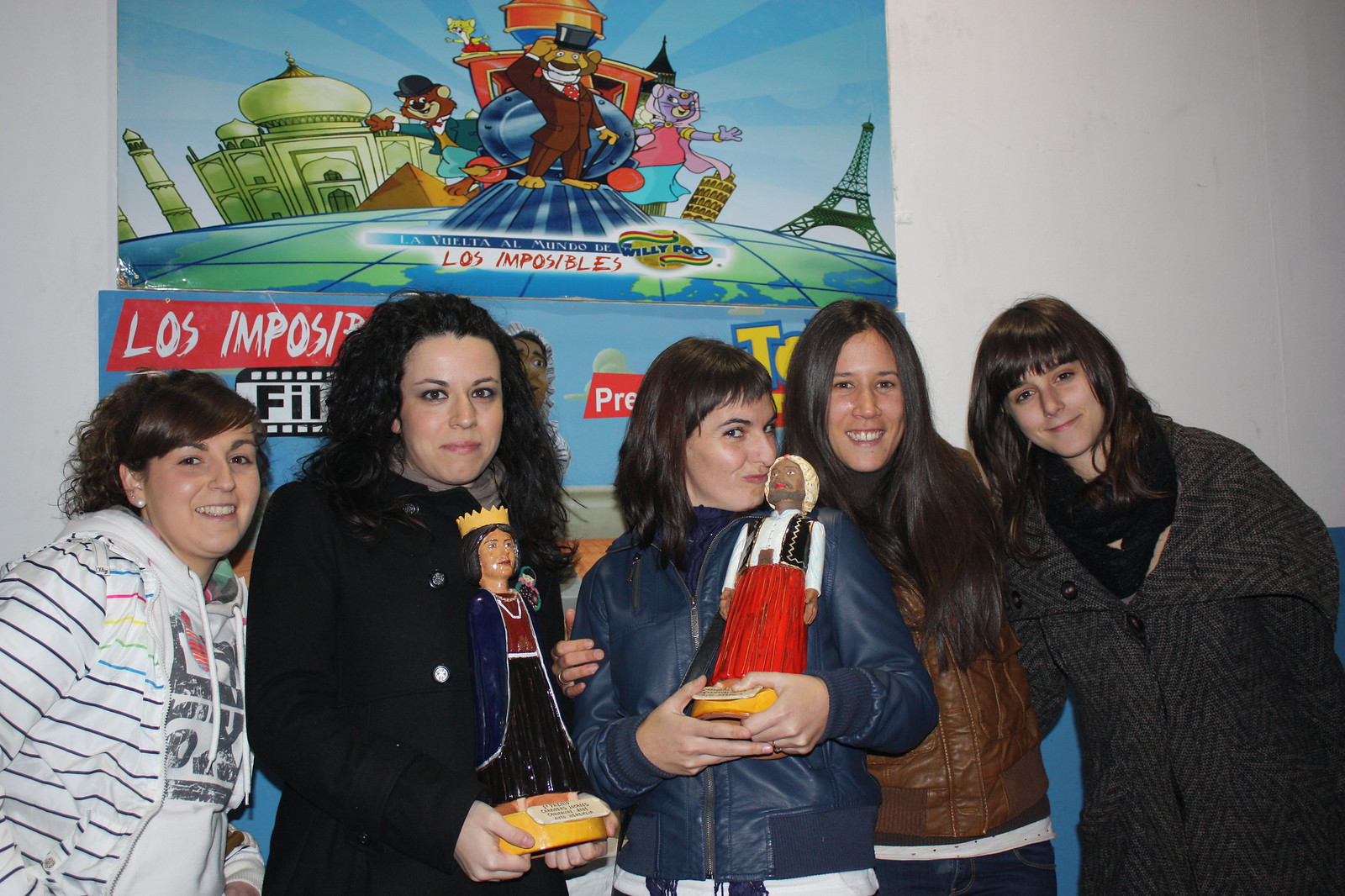This photograph features five young Caucasian women standing in a line in front of a wall featuring a poster of cartoon characters. All of the women have long, dark hair and are dressed in various styles of winter clothing. From left to right, the first woman has dark brown hair styled in a ponytail with straight hair in the front and curls in the back. She is wearing a white striped jacket over a white t-shirt. The second woman, with long black curly hair, is clad in a black jacket and is holding a statue of a woman wearing a crown. The center woman has dark brown hair and is dressed in a blue jacket, holding a statue of a South Asian man in a traditional turban and vest. The fourth woman also has long brown hair which falls below her chest, and wears a brown jacket. The last woman on the right has black hair just below her shoulders and is dressed in a gray jacket with a black scarf. Behind them, the poster showcases an array of animal cartoon characters positioned between stylized cartoon depictions of the Taj Mahal and the Eiffel Tower, with the text "Los Imposibles" at the top. The women are all looking directly at the camera, creating an engaged and cohesive group portrait.